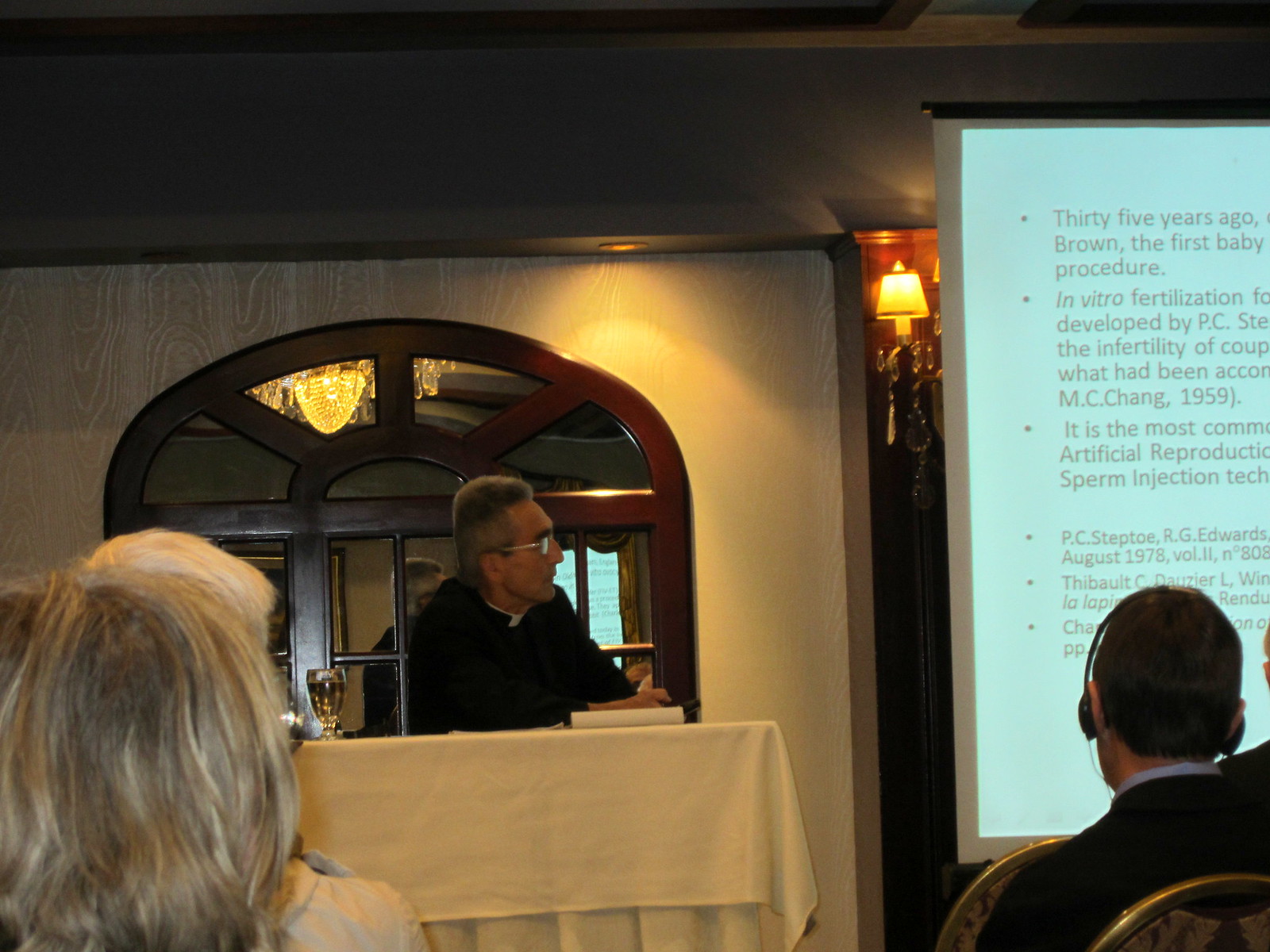The photograph depicts a priest standing at a table, identifiable by his white collar and glasses, delivering a lecture to a congregation. He is situated near a mirror with a dark wooden frame, which reflects the room's lit interior and a chandelier. On the table next to him is a glass of water. The priest is looking towards a projector screen on his left (our right), although the screen is partially cut off and only the beginning of the text is visible, starting with "35 years ago." The image is taken from the back of the room, emphasizing the audience. To the forefront, the back of a blonde-haired woman’s head is visible, alongside a man in a suit wearing headphones. Both appear to be attentive listeners, further highlighted by other individuals scattered throughout the seated congregation.